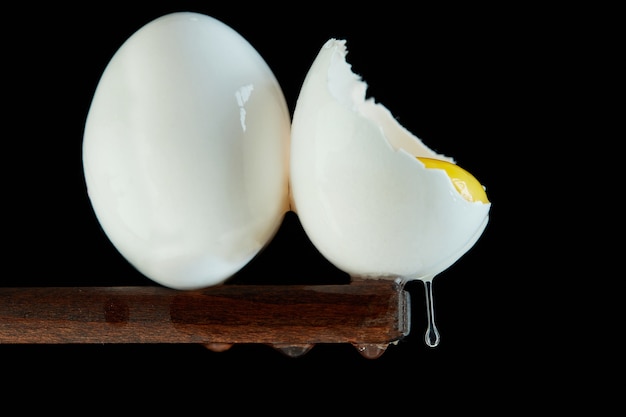The image depicts two eggs positioned on a dark brown, mahogany-like wooden stick that protrudes from the left side of the frame and extends toward the right. The background is completely black, emphasizing the eggs and the wooden surface they sit upon.

On the left, an intact, hard-boiled egg stands upright, with its shorter end facing up and reflecting a bit of light, giving it a shiny appearance. On the right, a cracked egg is split diagonally, creating jagged edges around its remaining shell, which forms a C-curve seat holding the yolk. The yellow yolk is visible and looks ready to spill over the edge, while some clear egg white has dripped down from the bottom, wetting the wood beneath it. This setup, viewed from the side, has a very artistic and deliberate arrangement, possibly intended for an art show or photography exhibit.